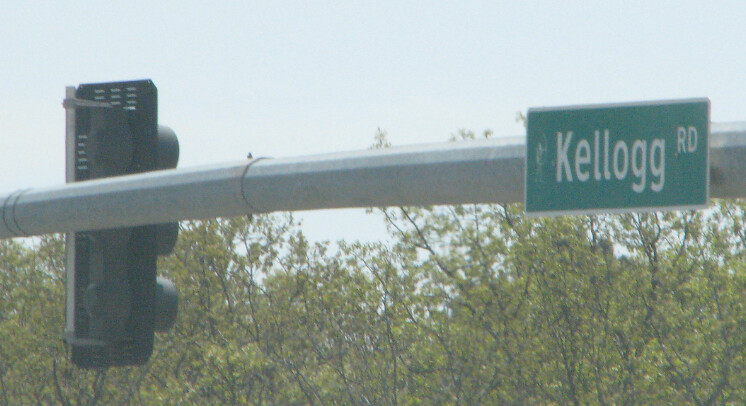This horizontal rectangular photograph, depicting a scene taken outdoors, captures a light blue sky adorned with brown tree branches and small green leaves, suggesting the transitional phase of early autumn. Prominently positioned in the center, a silver pole extends horizontally across the image, supporting a green street sign on the right and a vertical traffic light on the left. The green sign, bordered in white trim, clearly reads "Kellogg Rd" in white text. Adjacent to this on the left, the back of a black-framed traffic light is visible, revealing the three circular housings for its lights but not their colors. The overall atmosphere conveys a serene yet ordinary street scene, with the quiet presence of nature and essential urban elements coexisting under a calm, light sky.